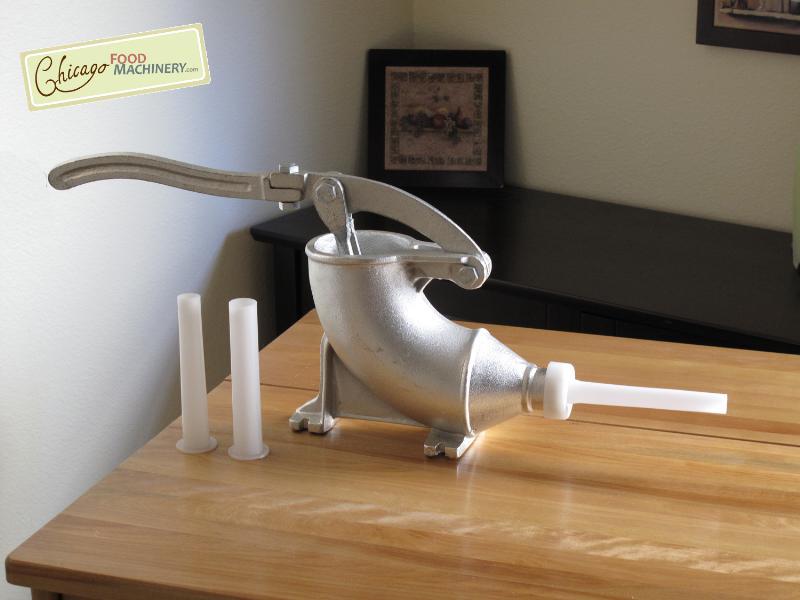The photograph captures an indoor scene featuring a vintage sausage stuffer machine prominently. The top left corner displays a yellow rectangle with the words “Chicago Food Machinery.com” emblazoned on it. The room’s walls are stark white, with a black-framed picture hanging on them. Against the wall is a black counter, which also holds a framed picture.

The manual sausage stuffer, likely made of cast iron and painted silver, rests on a light wooden countertop in the foreground. The machine consists of a large, curved metal tube reminiscent of a quarter-circle macaroni shape, and it features a handle used to press the filling through. This mechanism funnels the filling into a cone-shaped end where a plastic tip is attached. The tip molds the filling into a casing, ready for sausage making. Behind the machine are two additional white tubes, possibly extra casings or parts of the stuffer.